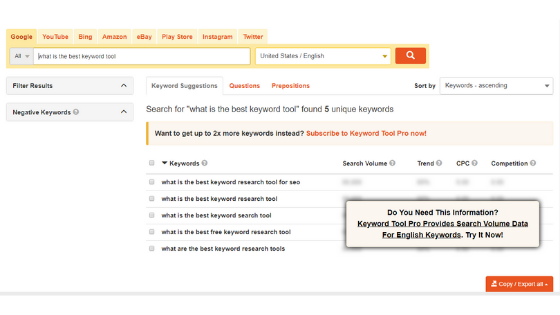This detailed image depicts a browser window themed in yellow hues, including the tabs and the address bar. The visible tabs from left to right are: Google, YouTube, Bing, Amazon, eBay, Play Store, Instagram, and Twitter, with the Google tab currently active. 

In the content area below the tabs, a search query is entered in a white search bar that reads "What is the best keyword tool?" To the right of this search bar are a language selection drop-down menu displaying "English / United States" and a prominent red search button.

The displayed webpage is organized into three tabs: "Keyword Questions," "Questions," and "Prepositions," with the "Keyword Questions" tab currently in view. The page title reads, "Search for 'What is the Best Keyword Tool' Found 5 Unique Keywords," with certain sections of the page grayed out to indicate inactive or disabled content.

On the bottom right of the browser window, a white box offers additional services with the text, "Do you need this information? Keyword Tool Pro provides search volume data for English keywords. Try it now." Directly beneath this box is a red button labeled "Copy / Export Mail."

Additionally, a "Sort By" drop-down menu is located on the page, showing the option "Keywords Ascending" as the selected sorting method.